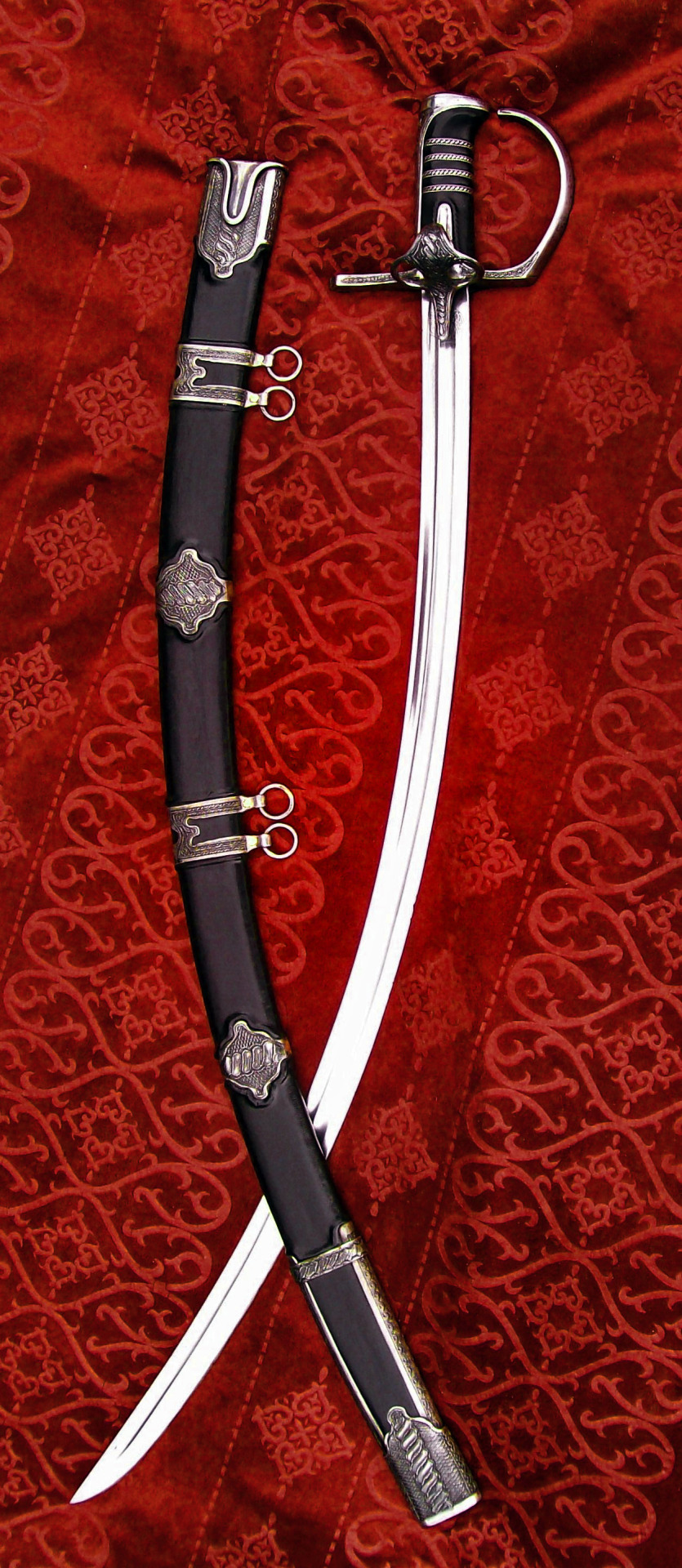This vertical photograph showcases an ornate, long, and slightly curved sword in its blackish-brown sheath, all set against a plush, richly designed red fabric that suggests a luxurious blanket or sheet. The gleaming, silver sword is thin and highly polished, not dull in the slightest. The sword and sheath are arranged parallel to each other, curving together at the bottom. The sheath features multiple metal accents and small handles or rings, including four holes grouped at the top and the center, possibly for attaching fabric to carry it over the shoulder. The sword’s handle is predominantly black with silver decorations and includes four noticeable stripes, and its hilt design hints at both functionality and historical aesthetic. This ensemble, reminiscent of an old-time samurai sword from perhaps the 17th or 18th century, elegantly highlights the intricate craftsmanship and historical allure of the weapon.